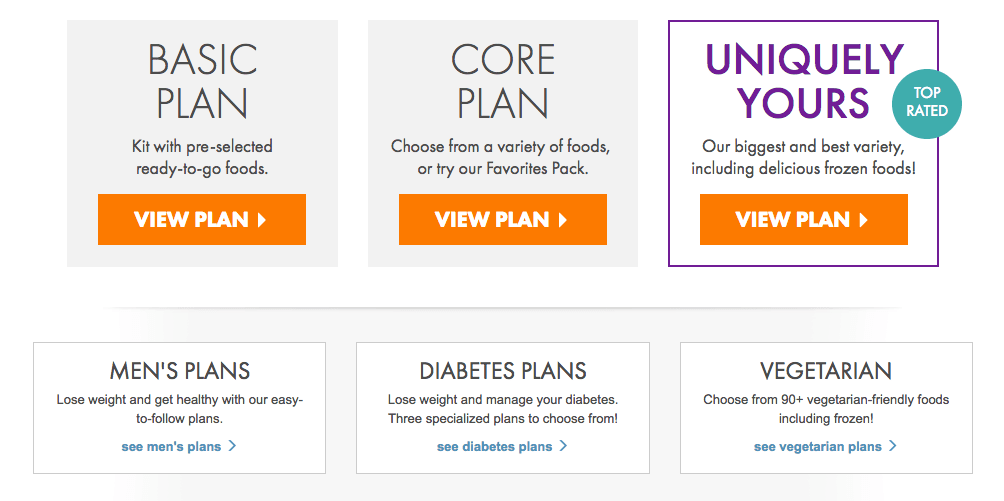The image shows a screenshot from a website featuring a comparison of different plans and categories. At the top, there are three squares with a gray background:

1. The first square is labeled "BASIC PLAN" in all capital letters, with "Basic" positioned above "Plan." Below this, it states, "Kit with pre-selected ready-to-go foods." An orange banner below has white text that reads "View Plan" with a right-pointing arrow.
2. The second square is labeled "CORE PLAN" in the same style as the first, offering the option to "Choose from a variety of foods or try our favorites pack." It also has an orange banner underneath with the same "View Plan" text and arrow.
3. The third square, titled "UNIQUELY YOURS," stands out with purple print and a purple border. It highlights "Our biggest and best variety including delicious frozen foods." Below this square is an orange banner that once again reads "View Plan" with a right-pointing arrow. Additionally, there is a small, round turquoise circle labeled "Top Rated" in white text on this square.

Below these top squares are three more sections, each consisting of a white square within a gray background:

1. The first square is titled "MEN'S PLANS" in all caps, with a link below that says "See Men's Plans" in lowercase blue letters and a right-pointing arrow.
2. The middle square is titled "DIABETES PLANS," followed by "See Diabetes Plans" with a right-pointing arrow in blue text.
3. The last square is labeled "VEGETARIAN PLANS," featuring a link that states "See Vegetarian Plans" with a right-pointing arrow in blue text.